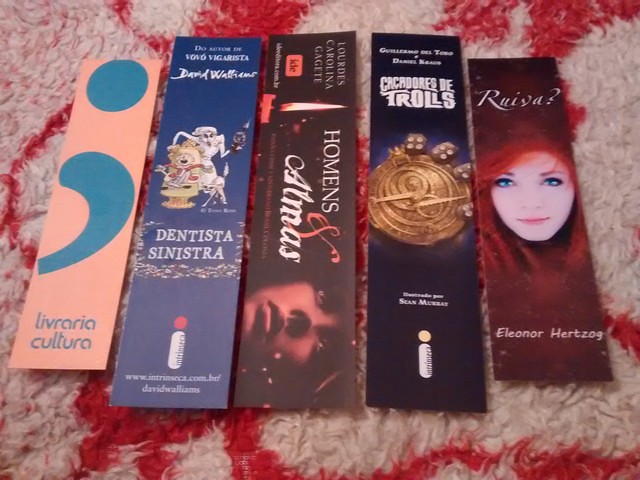The image showcases five rectangular bookmarks laid out on a dingy white rug with a red swirly pattern. The first bookmark stands out with a pink background featuring a blue semicolon and the text "Livraria Cultura." The second bookmark, set against a blue backdrop, has the title "Dentistas Intrista" and depicts cartoon characters. The third bookmark presents a gradation from black to red and features faint imagery, including a looming face. The fourth bookmark, displaying the text "Cacadores de Trolls," highlights a golden circle image and various dice. The final bookmark, set on a brown background, reads "Ruiva Eleanor Herzog" and portrays a pale woman with striking red hair and blue eyes. All the text appears to be in Spanish, and each bookmark features distinct illustrations and designs, contributing to a vivid, eclectic visual display.